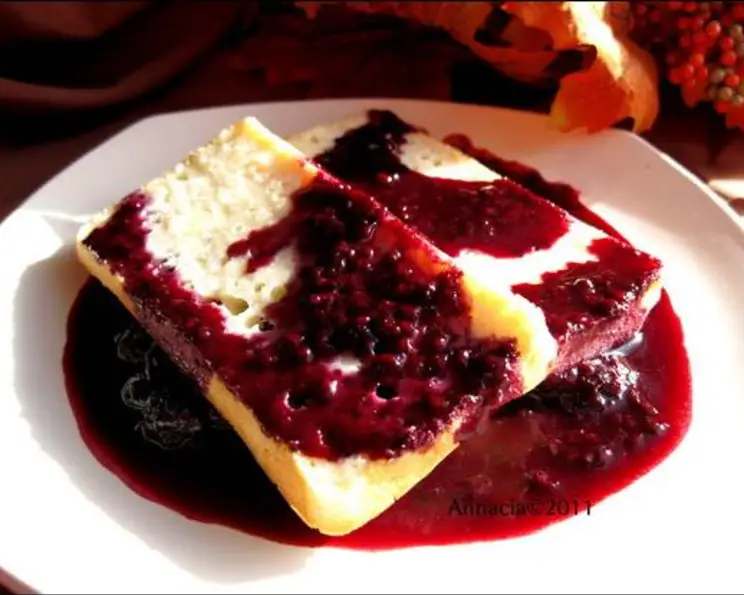The image depicts an appetizing dessert presented on a white plate, resting on a table. The centerpiece of the dessert is a piece of bread that's been sliced in half, displaying a creamy white interior with visible holes. The bread slices are partially covered and surrounded by a thick, deep red berry sauce, likely raspberry jam, featuring bits of berries that give it a syrupy texture. The rich, vibrant color of the sauce pools around the bread, creating an appealing contrast against the white plate. In the blurred background, a dark, orangey plate and some grapes with a grape leaf can be seen, adding depth to the image. Notably, the plate has a watermark that reads "2011" and possibly "on Asia," suggesting it might be showcasing a dish from either a culinary studio or a restaurant advertisement. This dessert is visually striking and promises a delicious treat.